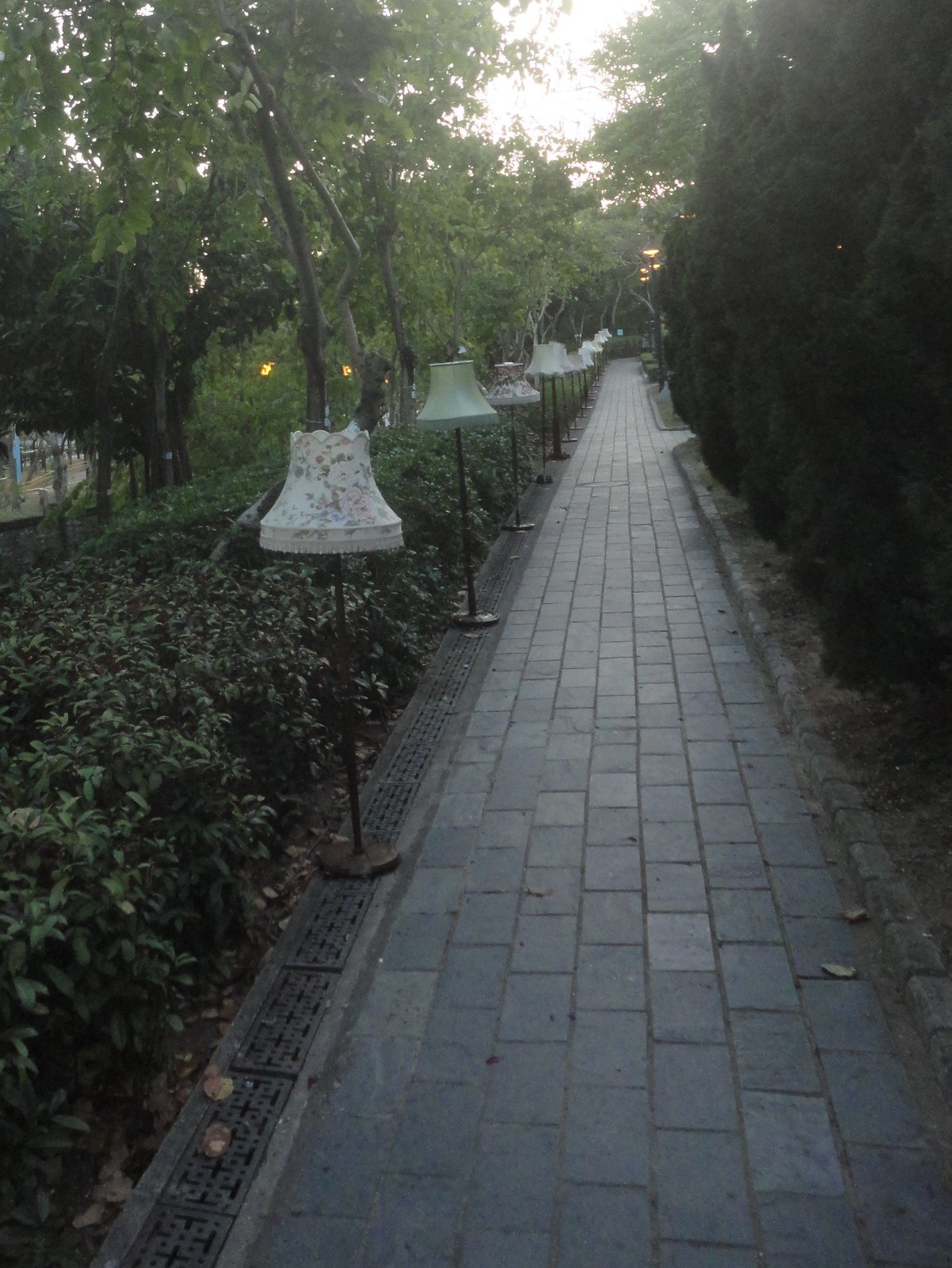The image depicts an outdoor scene featuring a long, gray brick pathway stretching from the bottom to the top of the photo. On both sides of the pathway, there are lush green plants and bushes, with tall trees in the background. The left side of the path is lined with numerous indoor-style standing lamps, each adorned with elegant old-fashioned white shades that feature floral decorations and tassels hanging around the edges. These lamps, perched on black stands, create a whimsical contrast to the natural surroundings. The sky, visible through the gaps in the foliage, appears grayish, suggesting that the photo was taken towards the end of the day. The pathway and its unique lamp decorations extend all the way from the foreground to the horizon, adding depth and intrigue to the scene.